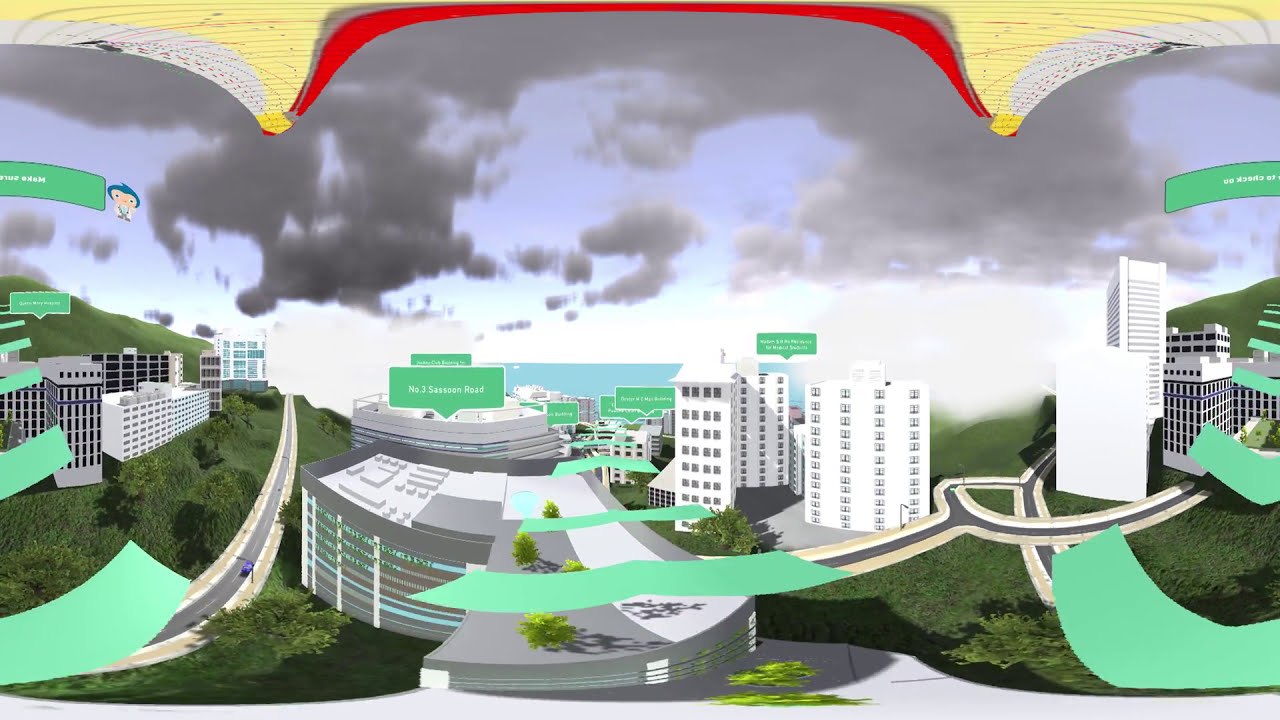In this computer-generated image, we see a detailed depiction of a sprawling neighborhood set against a landscape that includes a coastline in the distance. The lower half of the image is dominated by a collection of roads, gray and white residential buildings, office structures, and trees scattered throughout. Among these, prominent tall white buildings stand in the center alongside a larger white building to the right. Above many of the buildings are green signs with white text presenting location identifiers like "Number 3 Cezanne Road" and "Number 1 Sasson Road." The text on other green signs is too small to decipher. The image also features an icon of a peach-colored avatar with green hair, dressed in a white jacket, located in the top-left corner. The upper half of the image reveals a cloudy gray sky, with the overall scene slightly distorted, suggesting it might be part of a panoramic view. Splashes of blue indicate water in the background, highlighting the coastal setting. The green stripes scattered throughout the image add another layer of textual information and visual interest to the digital artwork.